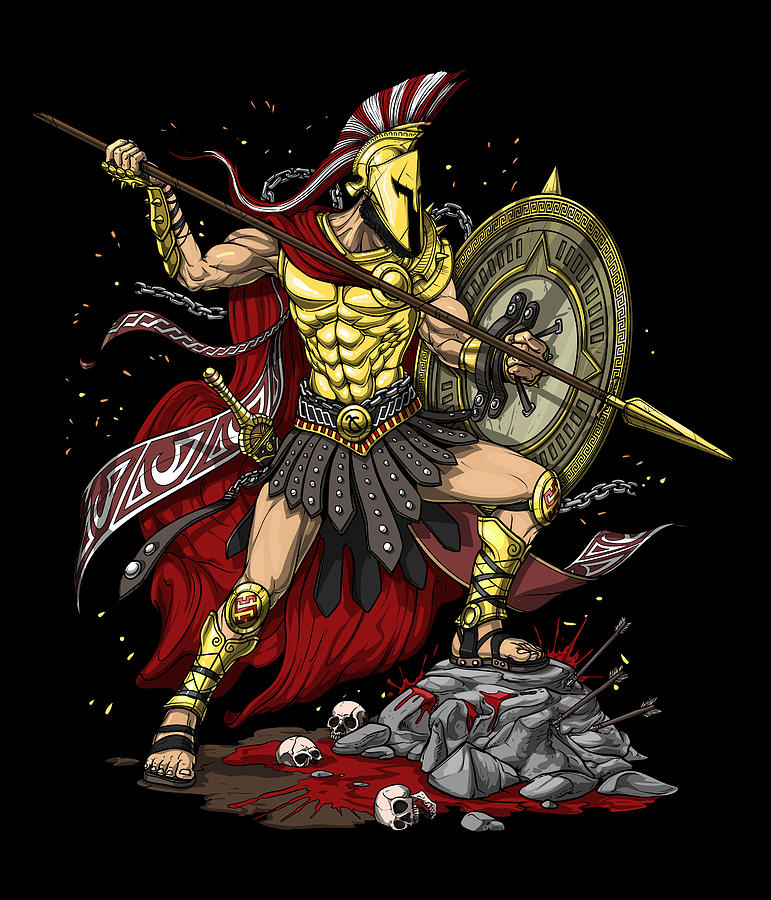The digital artwork portrays a highly detailed rendition of a Greek or Roman warrior, reminiscent of the Spartan King Leonidas. The warrior is adorned in golden armor, including a elaborately detailed chest plate that highlights exaggerated abdominal muscles, and gold shin guards with circular knee pads featuring red designs. He is also equipped with gold wrist gauntlets and a gold face mask, topped with a prominent red and white striped mohawk.

The warrior's attire is completed with brown sandals and a leather skirt, while a large red cape flows dramatically from his back. He is shown in a dynamic pose, with one leg propped on a pile of bloodstained rocks that are pierced with numerous arrows, and three skulls positioned at his feet, with blood flowing around them.

In his left hand, the warrior grips a large, round shield adorned with a lethal spike on top, while his right hand wields a long wooden spear tipped with a gold, triangular spearhead pointed to the right. Additionally, a sword is strapped to his back, hanging below his waist. The character is facing to the right, depicted in a state of readiness, as if defending or protecting himself. The entire scene is set against a stark black background, enhancing the dramatic and imposing nature of the warrior.